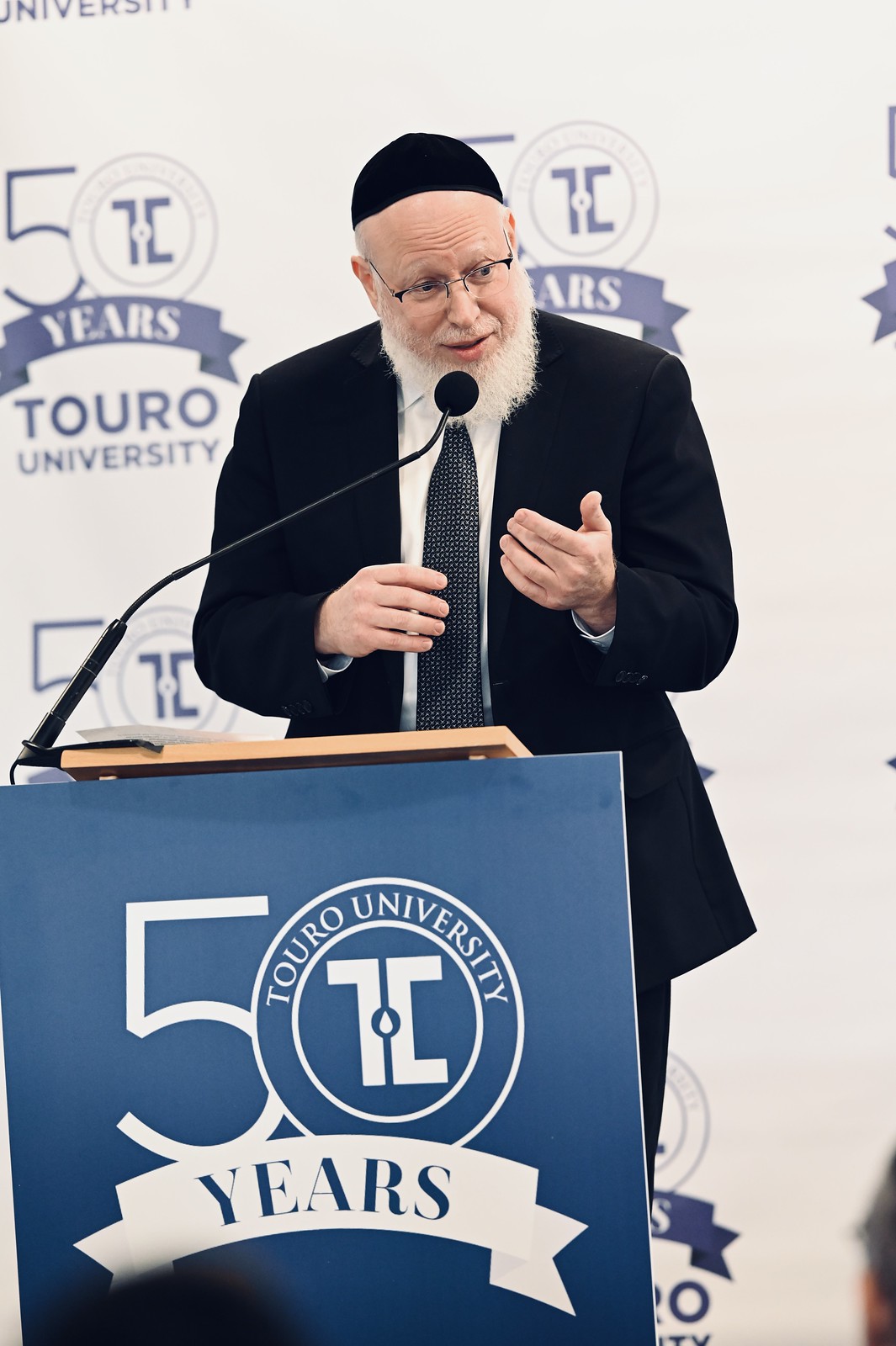The image features a distinguished man at a podium, dressed in a black suit with a white-collared shirt and a black tie dotted with tiny white spots. He sports a long white beard, glasses, and a black yarmulke. He is speaking and gesticulating with his hands, with a black microphone positioned close to his mouth. The podium is wooden and features a blue sign emblazoned with "50" in large white numbers, within the zero is the logo of Touro University, which includes a stylized "T" and a water drop symbol. Below this, in white text, it reads "Touro University" and "years." Behind him, draped against a white background, is a banner repeating "50 years Touro University" in blue lettering. This setup suggests a significant celebratory event, marking the university's 50th anniversary.